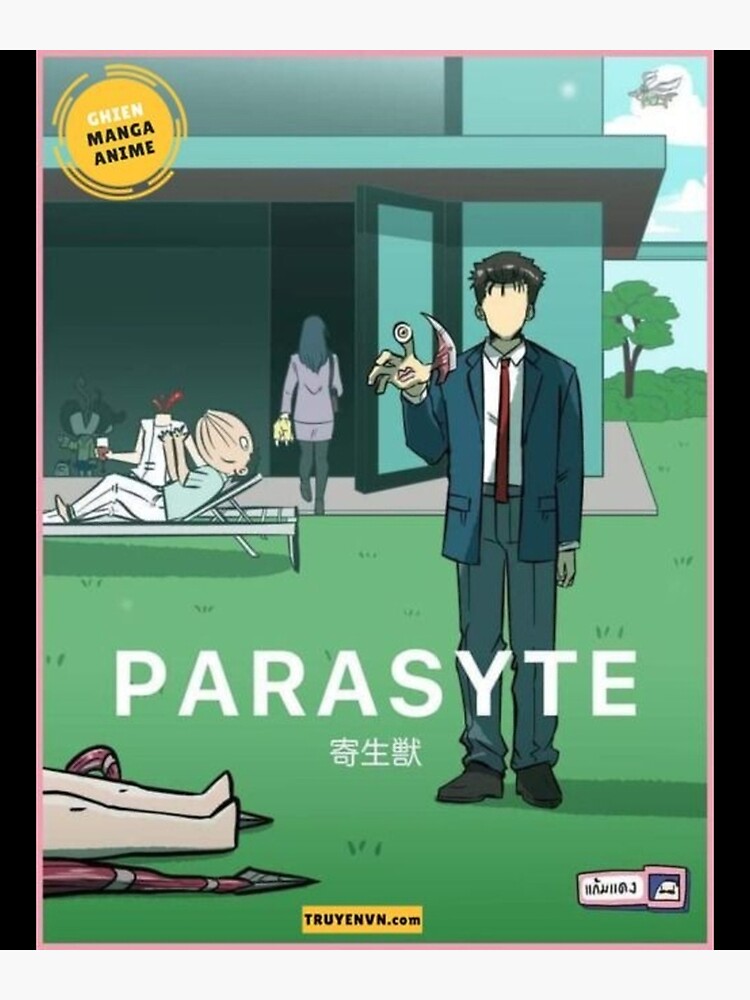The image appears to be a computer-generated cover for a graphic novel or manga titled "Parasite," with distinct elements reminiscent of the movie of the same name. At the top, the text "Chien Manga Anime" is displayed, accompanied by an unreadable symbol. The focus is on a faceless young Asian man who stands on the grass outside a large home. He’s dressed in a blue suit, red tie, and white shirt, with bluish-green pants and gray boots. His right hand is grotesquely mutated, featuring a blade on the thumb, an eyeball on one finger, and lips on the palm.

Nearby, a disturbing scene unfolds on a patio. A woman with a distorted, stretched-out face sits on a patio chair, while a headless person sits next to her. Another woman, who appears to have decapitated the person, walks into the building with the severed head. Additionally, at the bottom left of the image, only the lower legs and feet of another person lying on the ground are visible, next to some sort of swords. The bottom text reads "TRUYNVN.COM" and "Parasite" (stylized as "PARASYTE") followed by Chinese or Japanese characters.